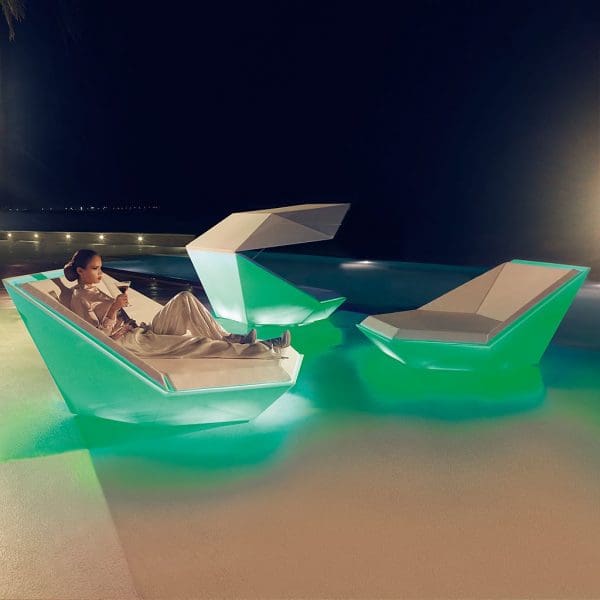In this futuristic poolside scene set against a dark night sky, a woman relaxes in one of three ultra-modern lounge chairs, artistically designed with geometrical shapes that resemble open mouths. These chairs feature green bottoms and brown tops and are arranged around a pool illuminated with soft blue lighting. The leftmost lounger has an awning for added protection, while the other two chairs face each other. The woman, dressed in a cream-colored, flowy outfit, is comfortably sipping a martini from a glass. The sleek, shiny metallic green floor beneath her enhances the modern aesthetic. In the dimly lit background, you can discern the contours of a pool, adding to the tranquil atmosphere of this outdoor night scene.